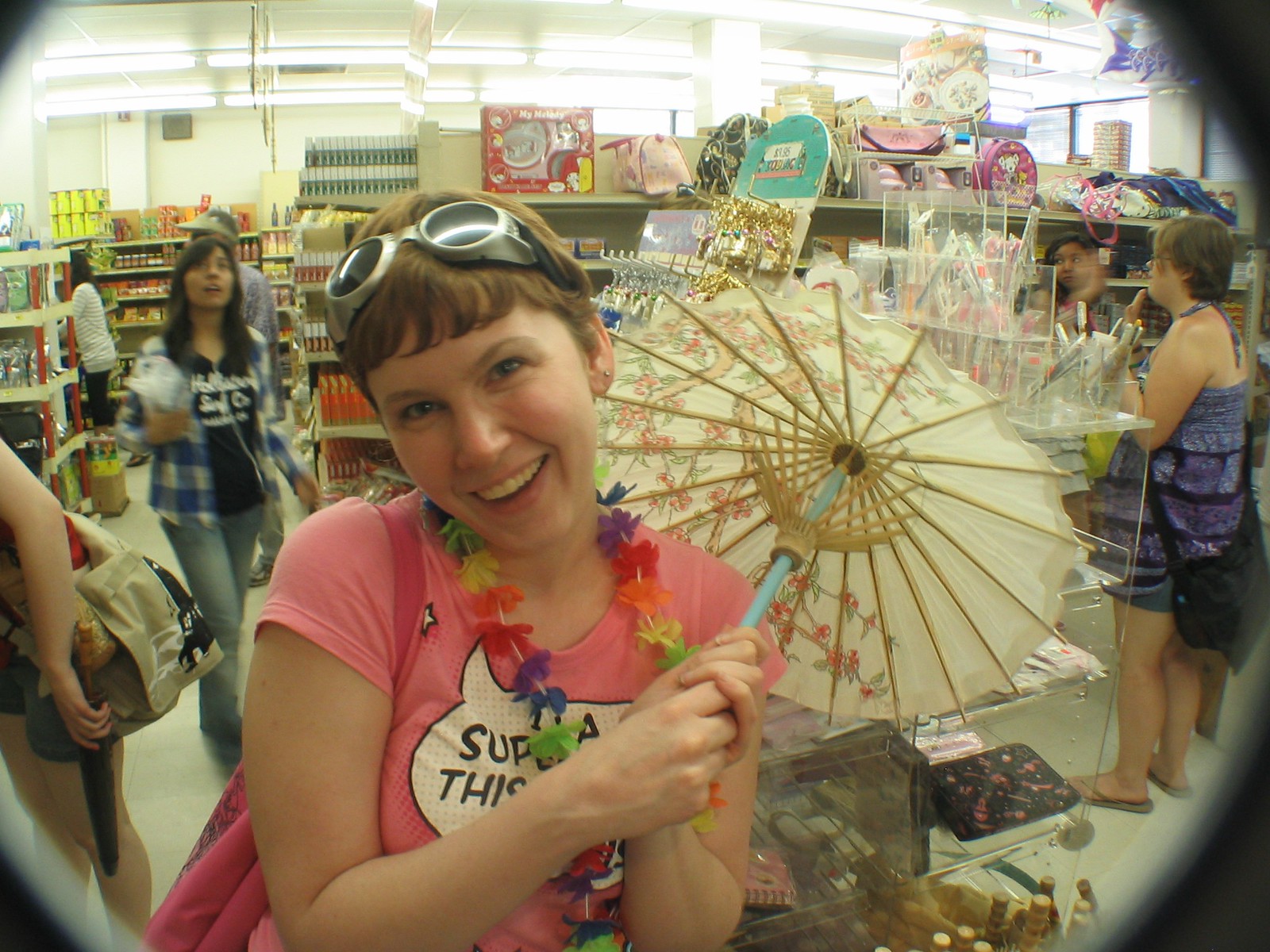This photograph features a light-skinned woman with a pixie hairstyle in a shade of strawberry blonde, standing in what appears to be a bustling department store that resembles a Goodwill or dollar store. She is smiling warmly, her head slightly tilted to the left, revealing her pixie upper teeth. She is dressed in a pink short-sleeved T-shirt with an indistinct white saying partially obscured by a multicolored garland of artificial flowers—purple, blue, orange, yellow, and green—that hangs around her neck. Atop her head rest white-framed sunglasses with dark lenses. 

In her hands, she holds a small decorative umbrella with a floral design, opened and placed over her shoulder. A pink-striped backpack is visible on her back. The background is lively with several people browsing shelves filled with a variety of products. One woman to her left is donning blue jeans and a shoulder bag, while another person with a brown book bag is partially exiting the frame. Another individual on her right wears a black shoulder bag and a short purple skirt, revealing their dark hair and shoulderless top.

The image, rectangular with curved blackened edges, gives a vignette effect, reminiscent of peering through a keyhole or peephole, framing this cheerful moment in the animated store setting.